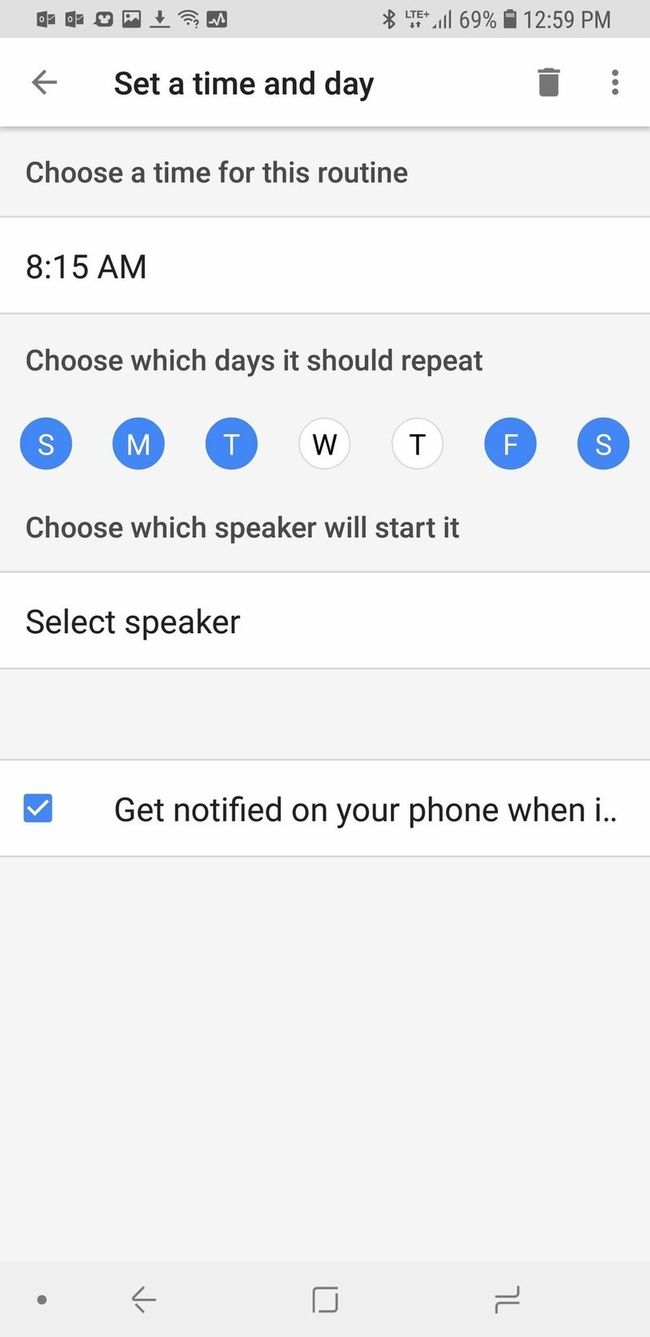The screenshot depicts the settings interface of an Android device. At the top of the screen, multiple notification icons are visible, including two identical icons resembling an envelope entering a square with a circle, a chat bubble featuring a Mickey Mouse head, a standard image icon, a download icon, a Wi-Fi symbol with a question mark, and a heart monitor icon. The device's Bluetooth is activated and it has full-strength LTE+ connectivity. The battery is at 69%, and the time displayed is 12:59 PM.

The settings screen details a routine configuration, prompting the user to set a specific time and day. The user has selected 8:15 AM as the desired time. The days Sunday, Monday, Tuesday, Friday, and Saturday are highlighted in blue, indicating they have been selected, while Wednesday and Thursday remain unselected in white. The interface also includes options to choose which speaker will start the routine and a checkbox to enable phone notifications.

The screen provides navigation options via a trash can icon, three vertical dots for additional settings, and a back arrow. At the bottom of the screen, standard Android navigation icons are partially visible, including a back arrow, a square, and additional overlapping squares, indicating recent apps.